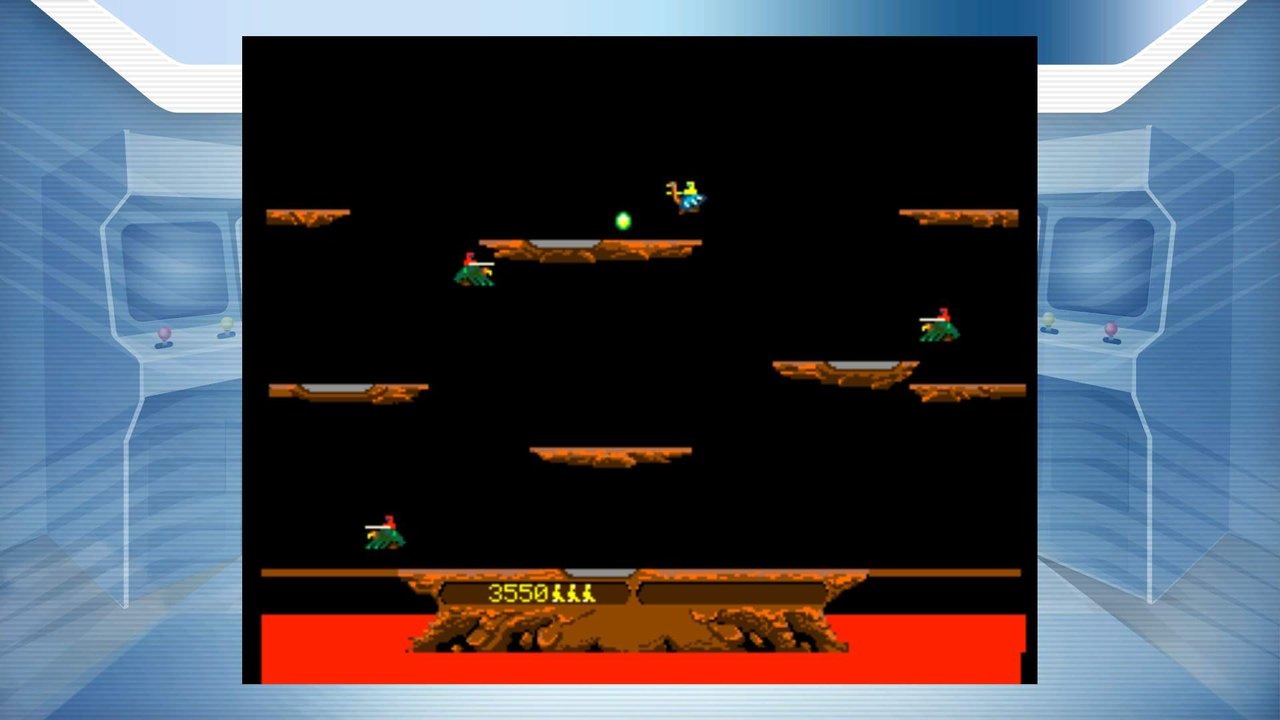This screenshot from what appears to be a modern retro-style video game closely resembles an 80s classic. The screen features a black background with brownish platforms, some adorned with silver spots. Floating mid-air are characters resembling jousting combatants, perched atop green, blue, and red-colored creatures, possibly pterodactyls or dragons. The characters include a yellow, Pharaoh-like figure, a green-and-red combination, and other vibrant hues. The score displayed is 3,550, indicating three lives left. The bottom platform holds the text "35550 person person person." The gameplay involves characters jumping across these platforms, collecting green eggs, and eliminating each other using found weapons, all while avoiding falling into the lava pits located at the bottom. The background simulates a simple 3D rendering of video game cabinets, complementing the retro aesthetic of the screen.